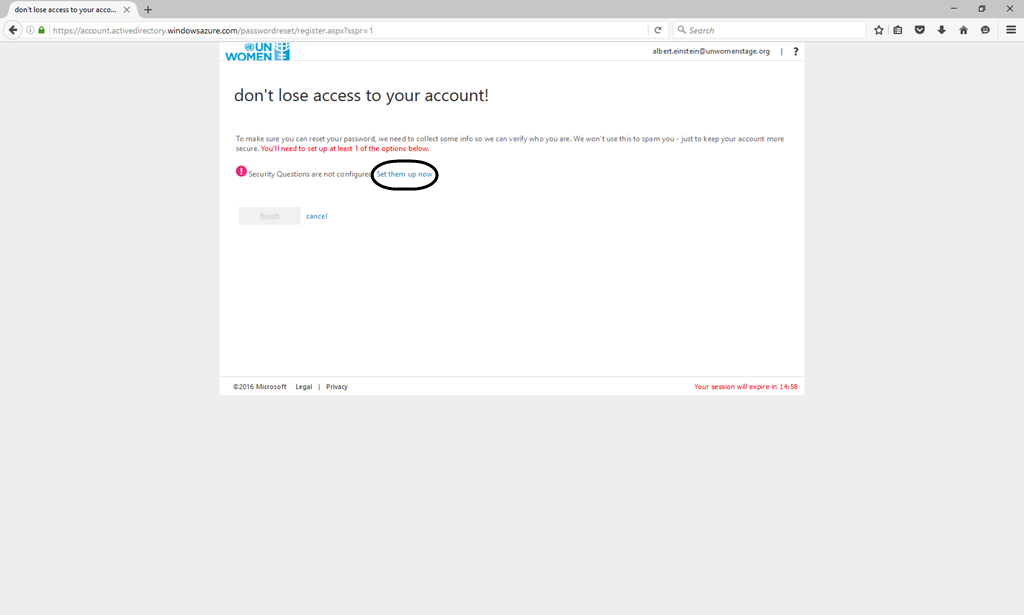Screenshot of a webpage featuring a gray interface with a top gray bar and a highlighted browser tab reading "Don't lose access to your ACCO...". Below this bar, the URL includes "WindowsAzure.com" and "password". The main content is a white rectangular box inset.

- **Top Left:** "UN Women" in blue text.
- **Main Heading:** "Don't lose your account!" with a small "d" at the front and an exclamation mark at the end.
- **Subtext:** "To make sure you can reset your password, we need to collect some info to verify who you are. We won’t use this to spam you, just to keep your account more secure."
- **Highlighted Notice in Red:** "You'll need to set up at least one of the options below."

Below this notice, there is a security warning indicated by a red circle with a white exclamation point stating "Security questions are not configured." Next to it is a blue link labeled "Set them up now," which is circled in red, seemingly marked by a tablet pen.

At the bottom of the box, there are two buttons:
- A gray "Finish" button.
- A blue "Cancel" link.

Finally, the footer reads: "2016 Microsoft Legal Privacy. Your session will expire in 14:58."